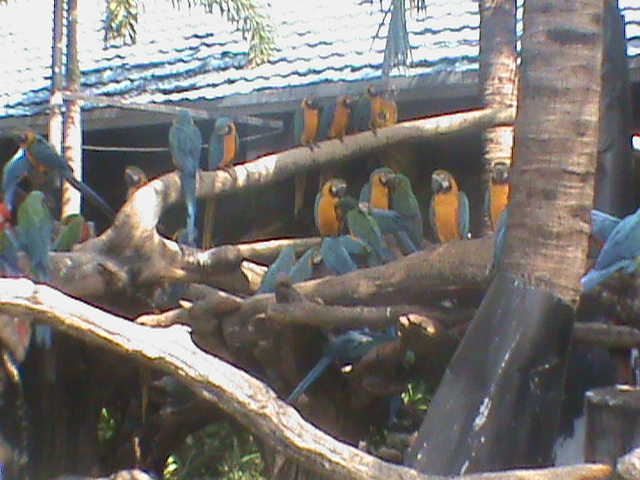This out-of-focus photograph captures a vibrant gathering of over two dozen parrots perched on a network of crisscrossing horizontal branches, set against the backdrop of a building with a gray Spanish tile roof. The majority of the parrots appear to be of the same species, featuring bluish-gray backs, bright yellowish-orange breasts and bellies, dark beaks with white facial markings lined in black. They also display some green on their necks and heads. The scene suggests an outdoor habitat, enhanced by the dappled sunlight filtering through overhead branches. Surrounding the area are several trees, including a couple of palm trees, and green plants visible near the ground level. In the lower right-hand corner, a shiny gray object can be seen. Overall, the image conveys a lively, semi-natural environment where these parrots roost and interact.